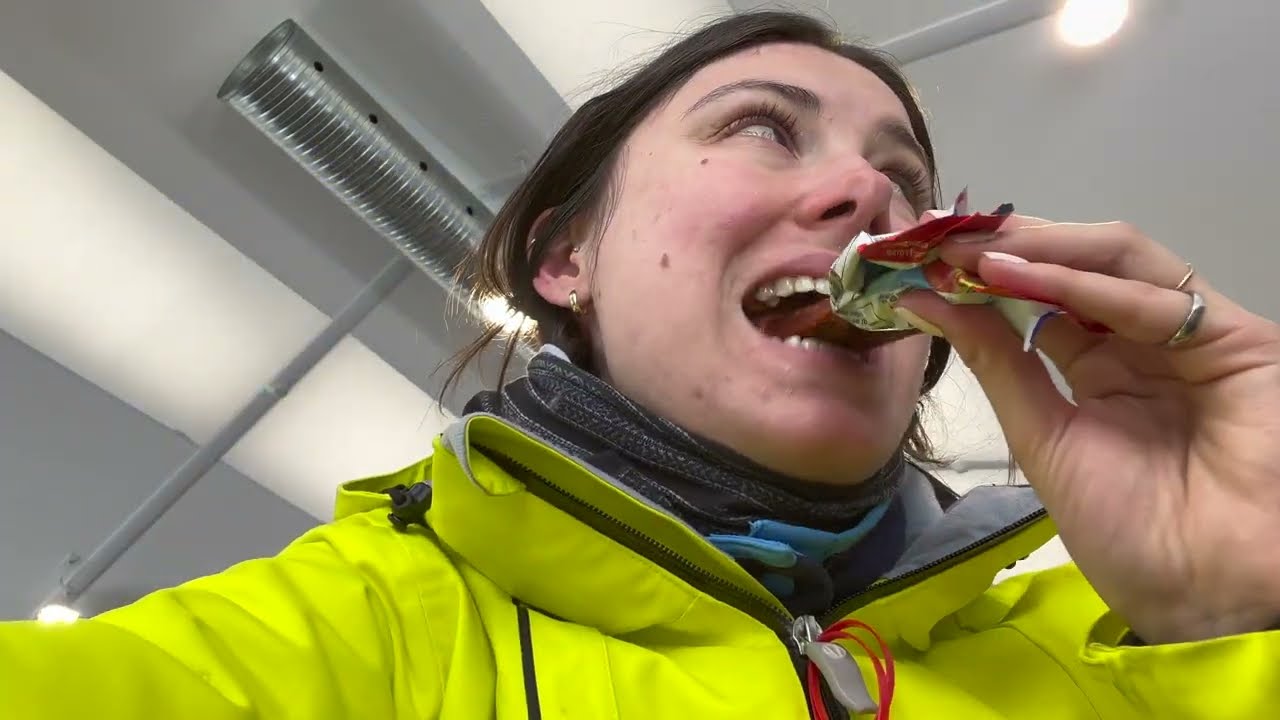This image is an upward-angled selfie of a woman with dark, pulled-back hair and tiny hoop earrings. She is wearing a vivid, bright yellow coat that zips up with a grey zipper, complemented by a scarf wrapped around her neck. Her face is slightly turned to her left, and she's caught mid-bite into a reddish nutrition bar, possibly a Laura bar, with its red and white wrapper partially visible. Her left hand, holding the bar, adorns rings—a silver one on her pinky finger and a thin gold band on her ring finger. Her eyes are brown, and she's looking away from the camera. The background reveals a clean-looking ceiling with exposed pipes, beams, and vents, indicating an industrial or modern setting.